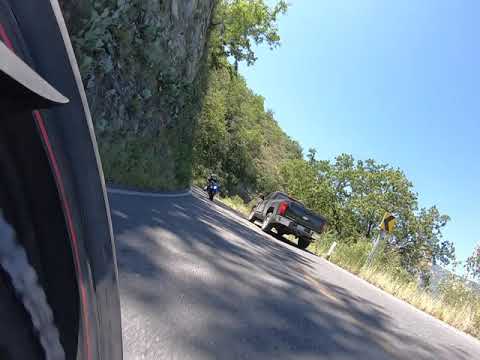The image captures a lopsided view of a well-maintained road under a sunny, clear blue sky, hinting that the camera might have been mounted on a motorcycle, positioned at an angle. In the foreground on the left, part of a reflective motorcycle wheel is visible, adding a sense of immediacy and perspective. The road curves around a steep stone wall adorned with shrubs and small trees, leading the eye towards a gray truck in the distance, its brake lights illuminated. To its left, a motorcycle is also in motion, trailing just behind the truck. On the right side of the road, there’s wild, unkempt grass and a sign indicating an upcoming curve. Further back, the landscape transitions into a grove of trees and more distant mountains.